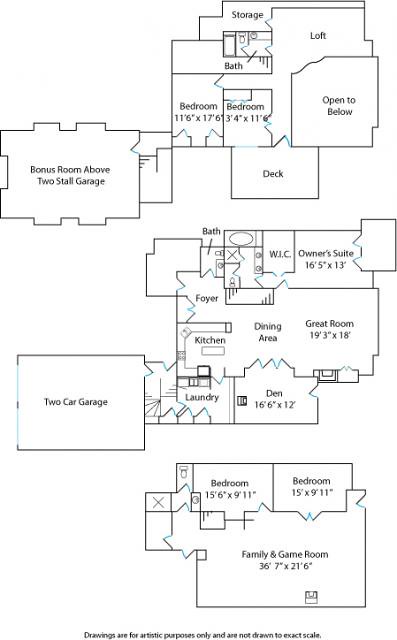The image depicts detailed floor plans for multiple buildings:

- **Top Floor Plan:**
  - **Storage Area:** Designated for storing items.
  - **Loft:** A versatile open space.
  - **Open to Below:** An area that is open to the level below, likely providing a view or connection between floors.
  - **Bedroom 1:** Measuring 3 feet by 4 feet by 11 feet.
  - **Deck:** A designated outdoor area connected to Bedroom 1.
  - **Bedroom 2:** Located below and to the left of Bedroom 1, measuring 11.6 feet by 17.6 feet.
  - **Bathroom:** Positioned above Bedroom 2, featuring space for a bathtub.
  - **Bonus Room:** Situated above a two-stall garage, providing additional flexible space.

- **Middle Floor Plan:**
  - **Bathroom:** Clearly marked.
  - **WIC (Walk-In Closet):** An ample storage space for clothing and accessories.
  - **Owner's Suite:** The primary bedroom suite.
  - **Great Room:** An expansive living area.
  - **Dining Area/Kitchen:** Combined space for dining and meal preparation.
  - **Den:** A smaller, versatile room.
  - **Laundry Room:** Designated area for washing and drying clothes.
  - **Garage:** A two-car garage for vehicle storage.

- **Bottom Floor Plan:**
  - **Two Bedrooms:** Located at the top of the floor plan.
  - **Family and Game Room:** Positioned at the bottom, providing space for family activities and recreation. 

The combination of these plans offers a comprehensive layout for living, storage, and recreational needs, detailed for practicality and convenience.